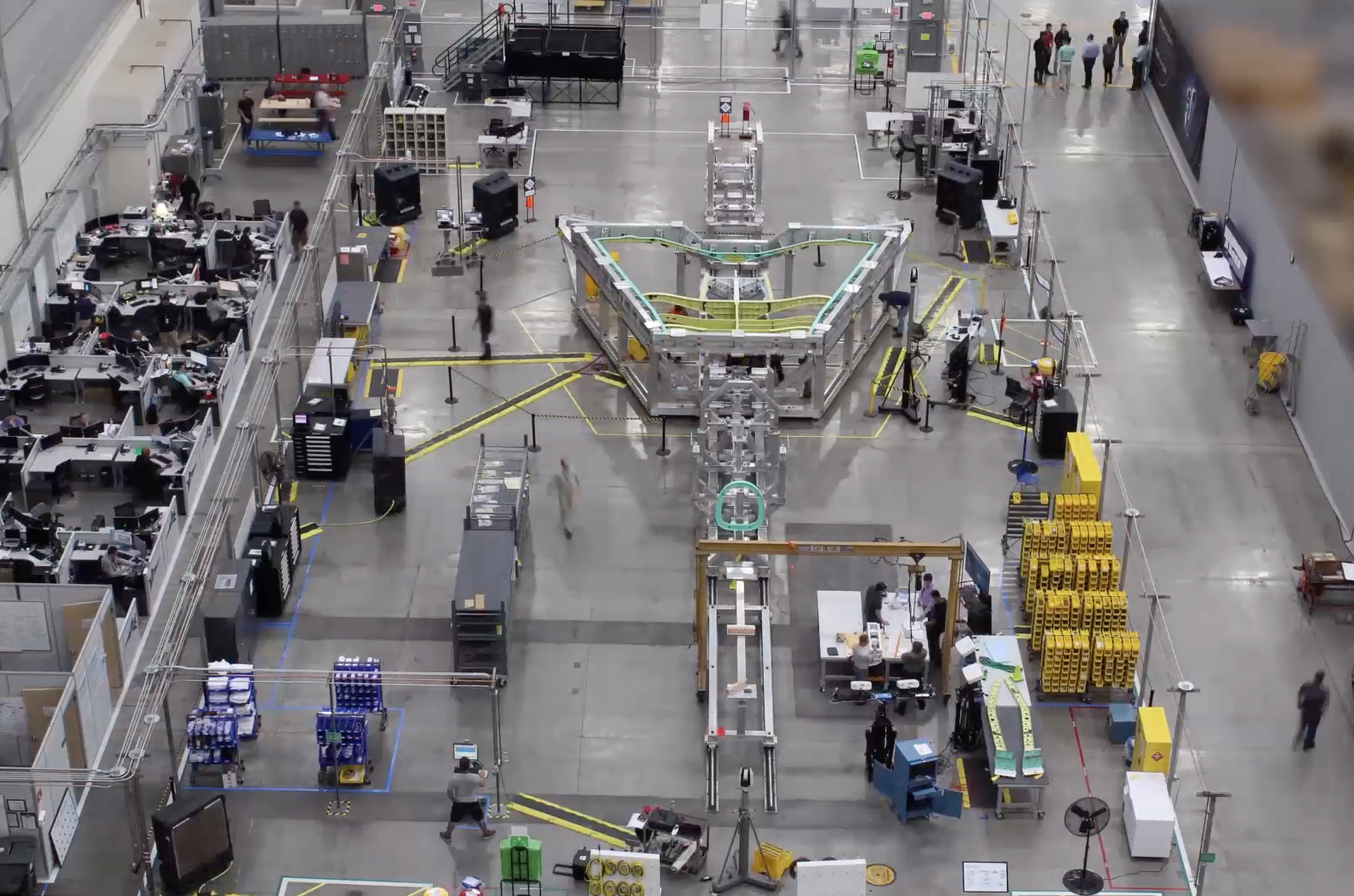This landscape-oriented aerial photograph captures a sleek, modern manufacturing floor. At its center lies a large, metallic structure resembling a column transitioning into a trapezoid, likely part of an assembly line for high-end manufacturing, possibly aircraft components given the aluminum-like frame. The floor, a clean, painted gray concrete, is organized with jigs, cranes, and yellow plastic dividers delineating various workstation areas. Industrial robots and machines are scattered throughout, emphasizing a technological and automated environment.

In the upper right corner, a group of men, appearing formal in suits, stand by, perhaps supervising or inspecting the operation. Additional workers are seen across the scene, engaged with computers and other tasks. On the left side, there is an office-like section with cubicles, desks, and conference rooms, seamlessly integrated into the factory setting. Various substructures and stored items also dot the area, while black cabinets and fans hint at the extensive support infrastructure in place. Despite the activity, no one seems actively working on the central structure, suggesting a shift change or preparation phase.